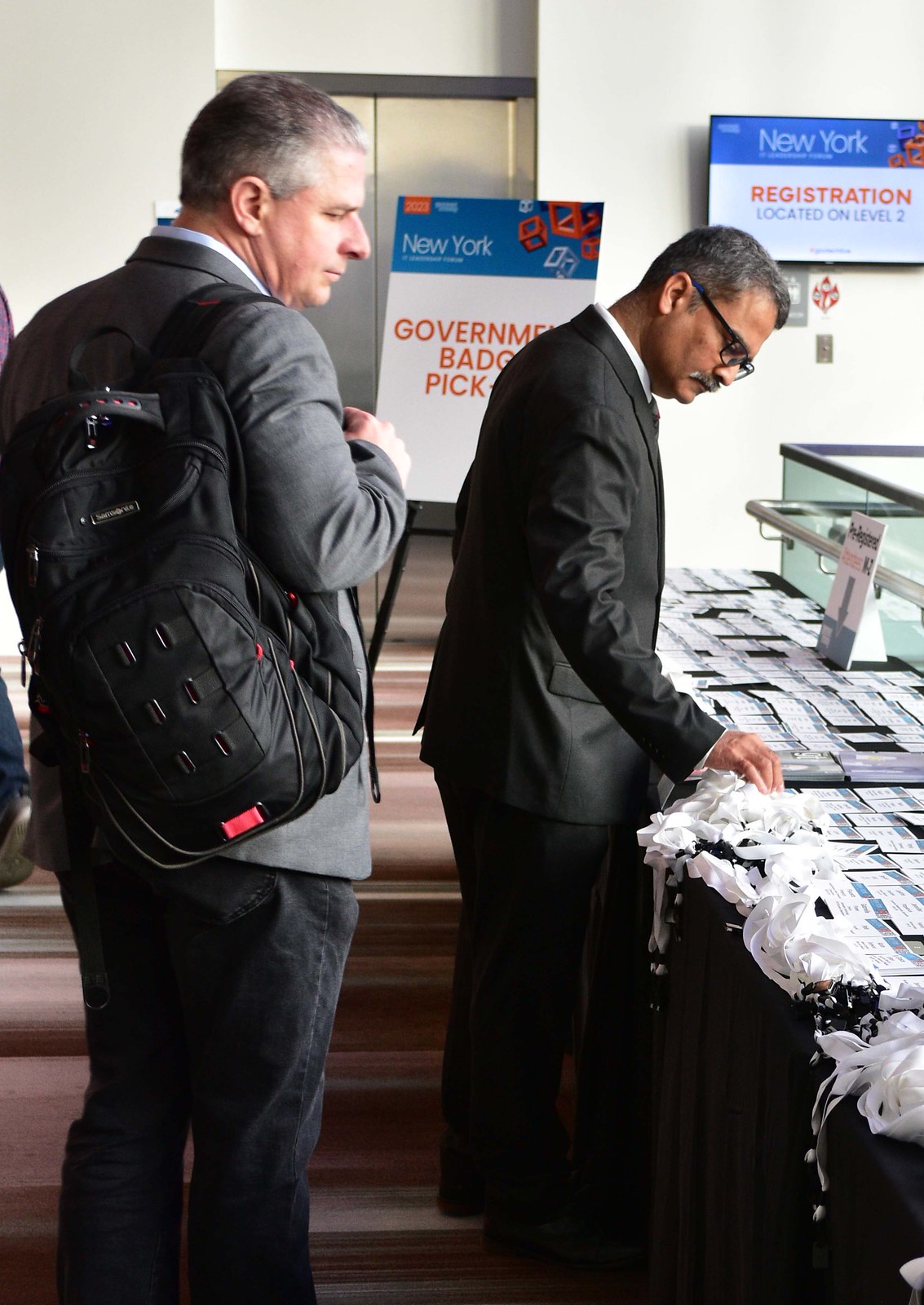In a bustling convention setting, two middle-aged men are seen engaging with a registration table, presumably in New York, as indicated by signage in the background. The man on the left, visible from his ankles upward, wears dark black denim pants, a gray business coat over a white collared shirt, and carries a large backpack over his right shoulder. Behind him, a sign reads "Government Badge Pickup," suggesting he might be waiting in line. To the right, another man, clad in a sharp black business suit, complete with black dress pants, a white shirt, a tie, and black glasses, is focused intently on the table. The table is draped with a black tablecloth and strewn with white lanyards and multiple small rectangular name badges. Both men appear to be in their 40s, with short gray hair, giving an impression of seasoned professionals possibly registering for a government-related conference. A TV on the wall and additional signage reinforce that the registration area is located on level three of the venue.